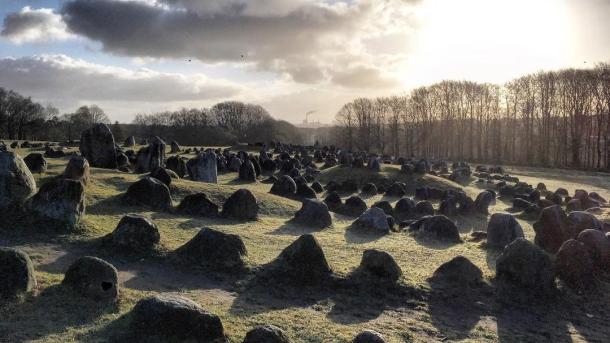The horizontal rectangular image depicts a sunlit outdoor scene of a harvested hay field, characterized by scattered yellowish debris from the harvester. Numerous round hay bales are strewn across the field, awaiting collection. The horizon reveals tall, leafless trees, suggesting it's late fall nearing winter. Above, a patch of bright blue sky is dotted with white clouds, and the sun gleams brightly in the top right corner, enhancing the clarity and brightness of the scene. The ground is dotted with some round boulders and rocks, adding texture to the landscape. There are no people or vehicles in sight, making the natural setting the focal point of the image.